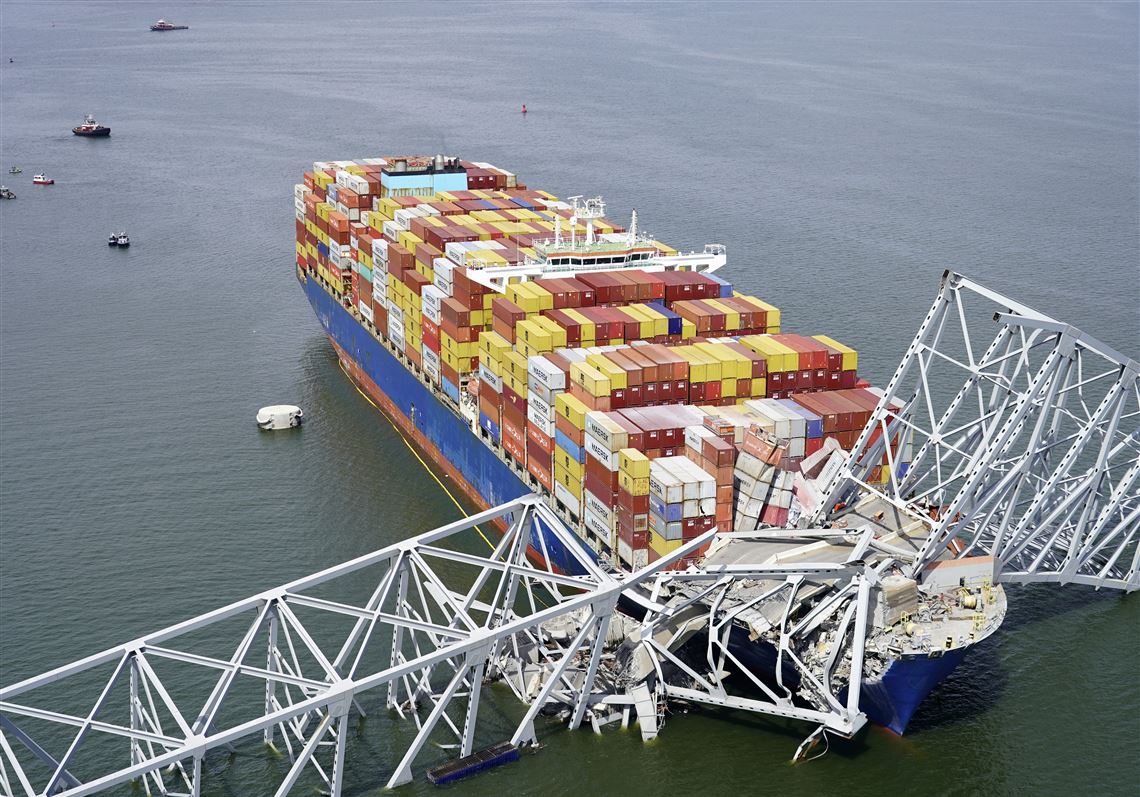The image depicts the dramatic aftermath of a major accident involving a massive shipping container vessel and a bridge. The ship, which has a blue and red striped hull, is laden with a multitude of brightly colored storage containers—white, blue, red, orange, and yellow—stacked high upon its deck. The scene captures the moment where a towering metal bridge, described as having a white frame, has collapsed onto the front of the ship, its twisted and torn sections resting heavily on the bow. The bridge's structure has smashed into the ship, creating a chaotic sight of metal and debris. Surrounding the scene are smaller rescue boats navigating the deep bluish-green waters, with personnel assembled on the bow of the ship, likely searching for survivors. The image is striking in its portrayal of scale and destruction, with parts of the bridge laying across the massive vessel and giving the impression that the ship might be grounded in the shallow waters.